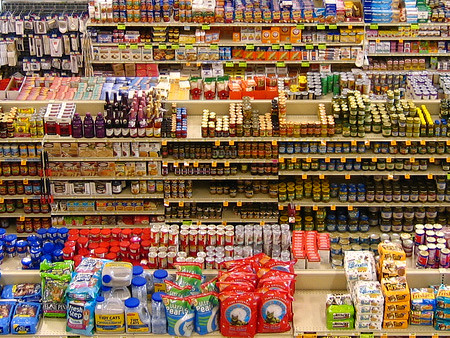The image presents an overhead perspective of a grocery store aisle, slightly wider than it is tall. The scene captures three distinct aisles, extending into the distance. The shelves, predominantly tan in color, rise to a height of six or seven units. In the foreground, an assortment of Tidy Cat cat litter dominates the pet aisle. Progressing deeper into the image, the second aisle appears to be stocked with various canned goods, potentially including pickles and other condiments. The furthest aisle, characterized by a predominance of red jars, suggests it might contain products like spaghetti sauce. Throughout the aisles, numerous yellow price stickers are visible, especially in the nutritional section that features a diverse range of bottles in green, brown, and black hues. The view, although comprehensive, is slightly distant, making some details less distinct but offering a broad overview of the store's layout and product variety.